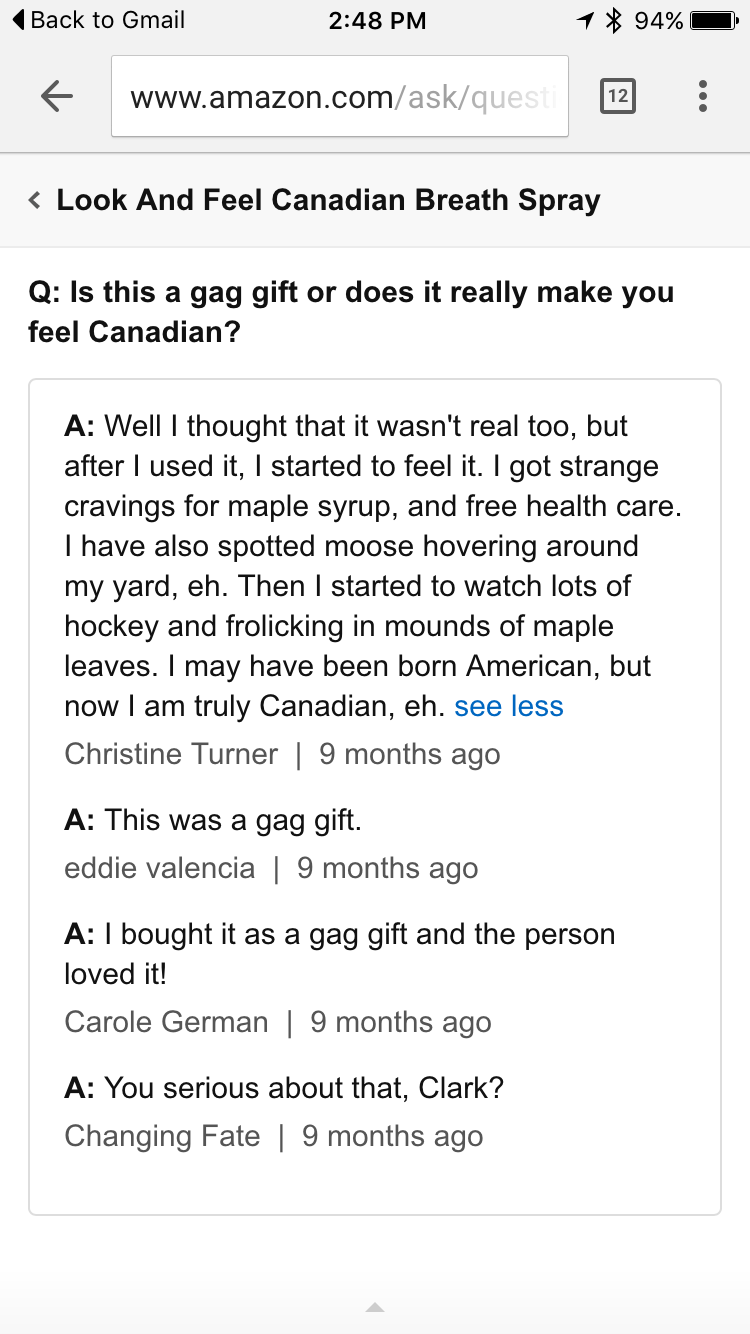This image is a detailed screenshot from the Q&A section of a product listing on Amazon. The screenshot primarily features a white background with a gray outline box containing four user answers to a question. The question, marked with a bold "Q:", asks, "Is this a gag gift or does it really make you feel Canadian?" The users' responses are indicated by a bold "A:" followed by their respective answers.

Above these answers, a ribbon element in light gray includes a back arrow and the label "Look & Feel Canadian Breath Spray." Above this ribbon, the typical iPhone or Android internet browser URL area is visible, showing part of the Amazon URL: "amazon.com/ask/question," which is truncated. The top of the screen provides additional contextual information: it’s 2:48 PM, the battery is at 94%, Bluetooth is connected, and there are 12 open browser tabs as indicated by a gray box with the number 12 next to the URL.

Each user answer includes the username of the person who provided it, separated by a line and the timestamp indicating that all responses were given nine months ago. The users who provided answers are listed as Christine Turner, Eddie Valencia, Carol German, and Changing Fate.